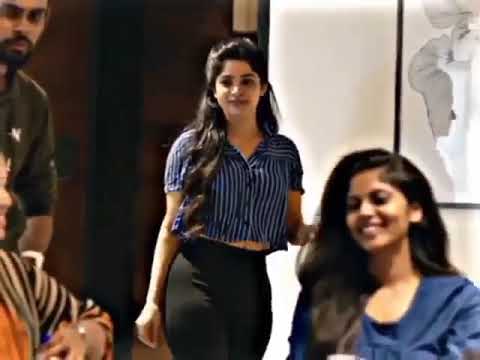The image depicts a vibrant scene featuring four individuals: two women on the right and two men on the left. The woman in front, seated and smiling warmly, is wearing a blue long-sleeve shirt, with her long black hair cascading down. She appears to be enjoying a cup of coffee, partially visible on the table in front of her. Standing behind her is another woman donning a blue and white vertical striped shirt that exposes a bit of her midriff, paired with black tight pants. Her long black hair extends all the way to her waist.

On the left-hand side, a man in a green long-sleeve shirt with a black beard stands with a serious expression. Partially cut off from the image is another man, noticeable by his brown and white striped shirt, of which only his arm and a portion of his face are visible. The background features what looks like a map or a white rectangular picture on the wall, contributing to the overall cozy atmosphere, illuminated by natural daylight.